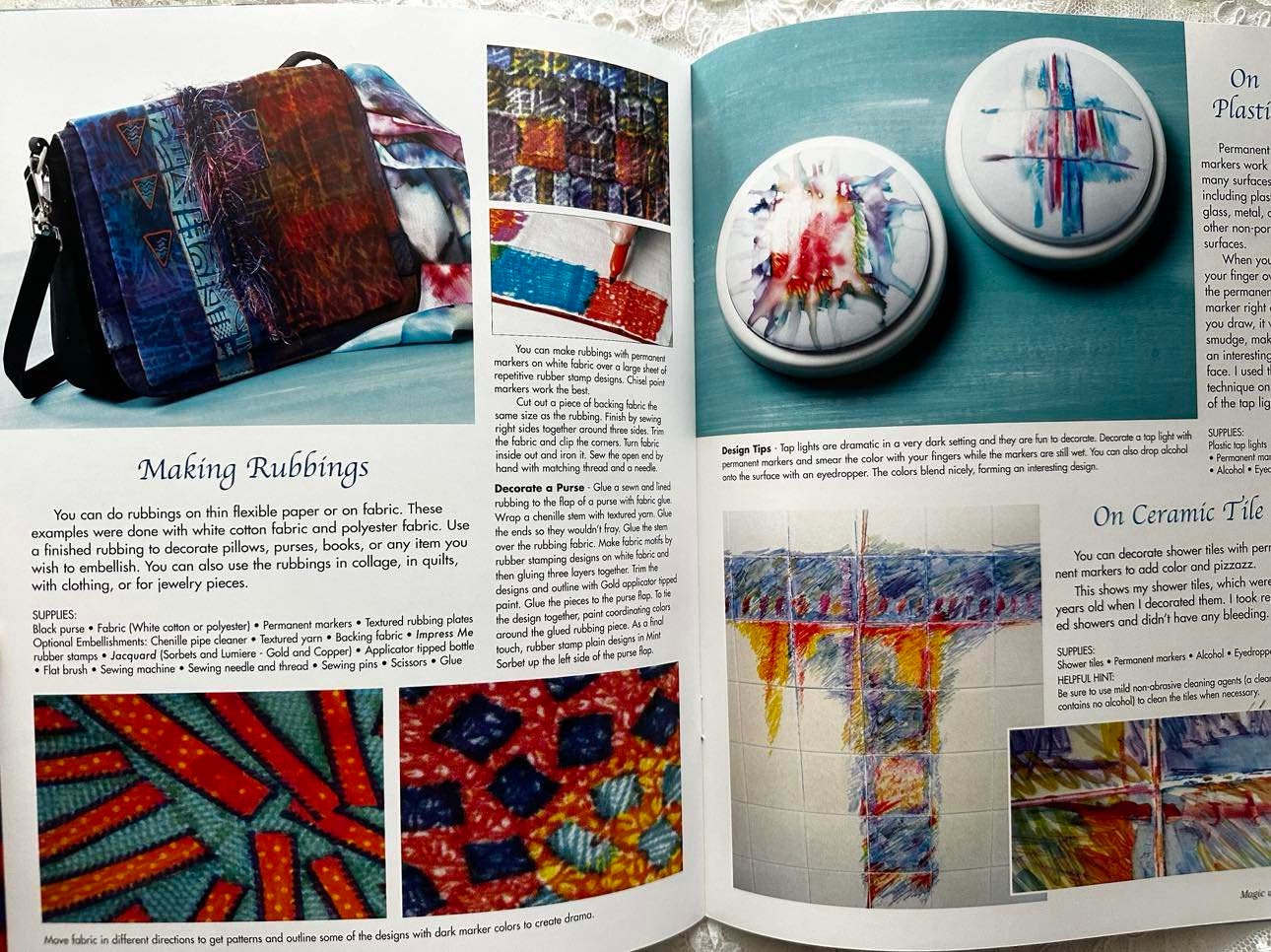The image depicts an open craft book, primarily focused on the technique of making rubbings. The book occupies most of the frame, with a delicate, white-patterned tablecloth visible in the background. The left-hand page showcases a multi-colored purse, transitioning from blue to purple to red, with captions indicating "making rubbings." Below this, there are two smaller images: a red square with a green border and a yellowish, scribble-like patch featuring black and bluish blocks. The right-hand page provides detailed instructions for creating rubbings on various surfaces, including plastic and ceramic tiles. Featured images include two circular objects with red and blue designs, and a ceramic tile with a white and blue-yellow pattern. The text is black, accompanied by vibrant, colorful photographs illustrating the outcomes of the rubbings, making the book both informative and visually engaging.